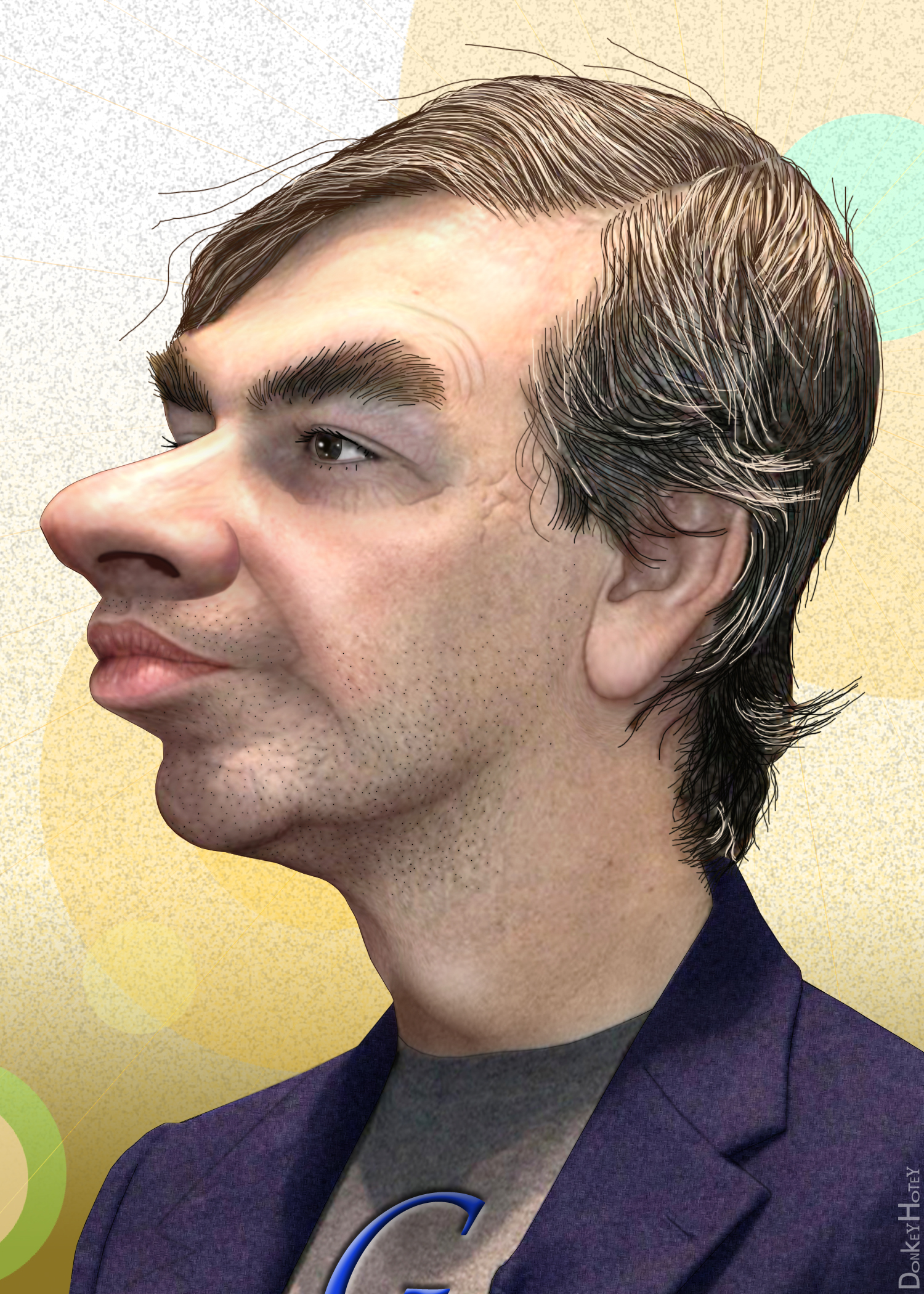The image is a heavily edited caricature of a man visible from the shoulders up. He wears a blue business coat over a gray graphic t-shirt, emblazoned with a large blue letter G with a black border. His face is exaggerated with a very large nose, almost no neck, and very large ears. His hair, a mix of black and white (salt and pepper), is short and combed over from the left side, with some spiky, slightly unkempt strands. His eyes and eyebrows are brown and bushy, respectively. He's facing towards the left with noticeable pink lips and a five o'clock shadow, complemented by wrinkles above and below his eyes. The watermark in the bottom right corner reads "DONKEY-HOTEY" from bottom to top, indicating a playful reference to Don Quixote. The background features swirls of yellow, green, white, light blue, and peach, adding to the whimsical nature of the image.